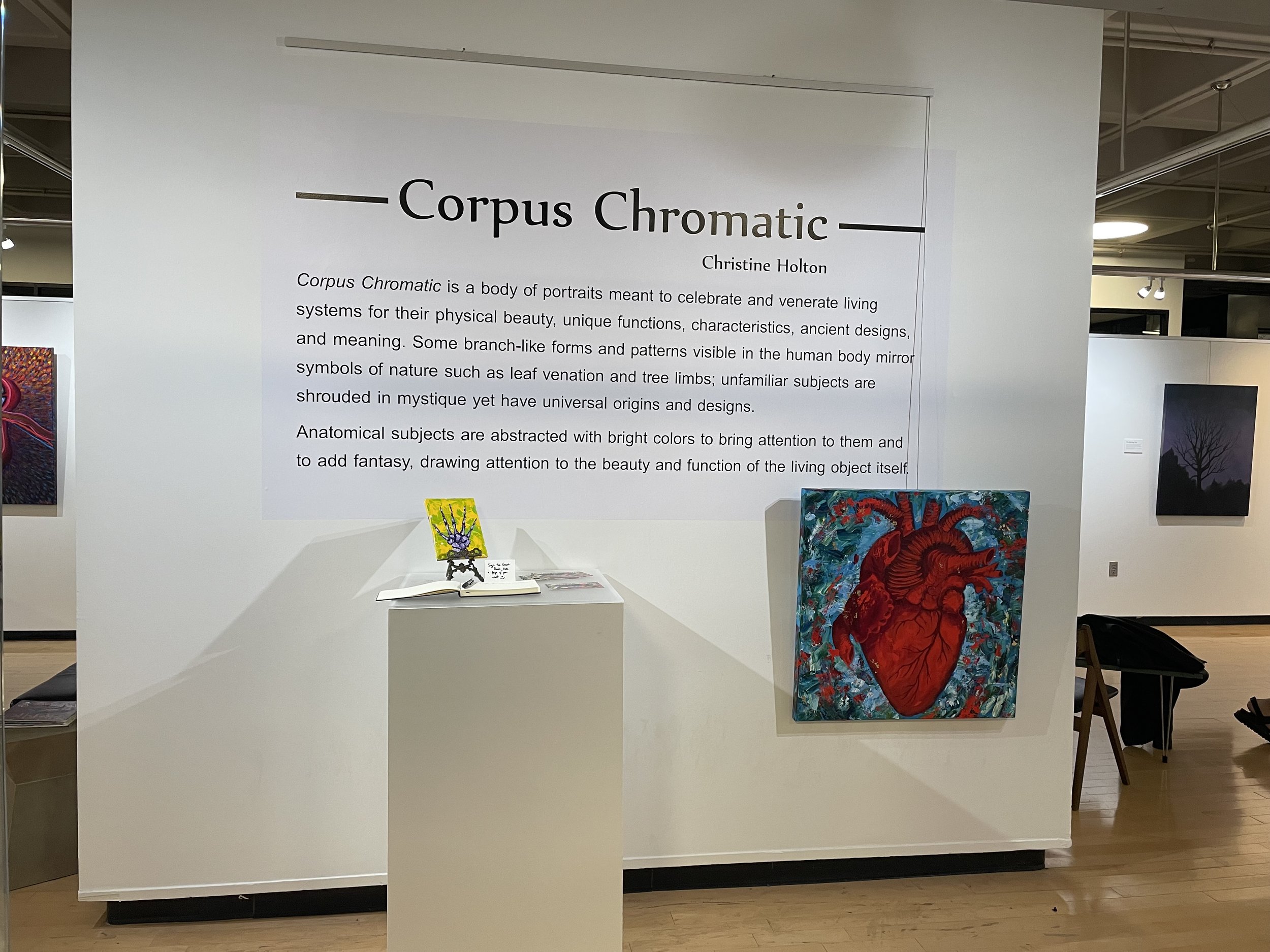The photograph depicts an art gallery exhibit titled "Corpus Chromatic" by Christine Holton. The gallery features high steel rafters and strategic lighting illuminating various artworks in the background, though they are not distinctly visible due to the distance. Dominating the foreground is a large white panel, approximately 10 feet high, that introduces the exhibit. The text on the panel explains the theme of "Corpus Chromatic," emphasizing its focus on celebrating living systems for their physical beauty, unique functions, characteristics, ancient designs, and meaning. The artist draws parallels between human anatomy and nature, using bright colors to turn anatomical subjects into abstract works of art.

Adjacent to this text is a striking painting of an anatomically accurate human heart rendered in vivid red hues, set against a blue background that resembles natural, plant-like patterns akin to stained glass. The pale blonde wooden floor of the gallery adds a warm contrast to the cool tones of the artwork, and a table stands nearby with pamphlets and a guest book. In front of the exhibit, various objects, likely part of the display, are arranged on what appears to be a rectangular podium with a yellow photograph that resembles an open book. A folding chair is positioned at the back of the exhibit, suggesting a space for observers to sit and contemplate the art.